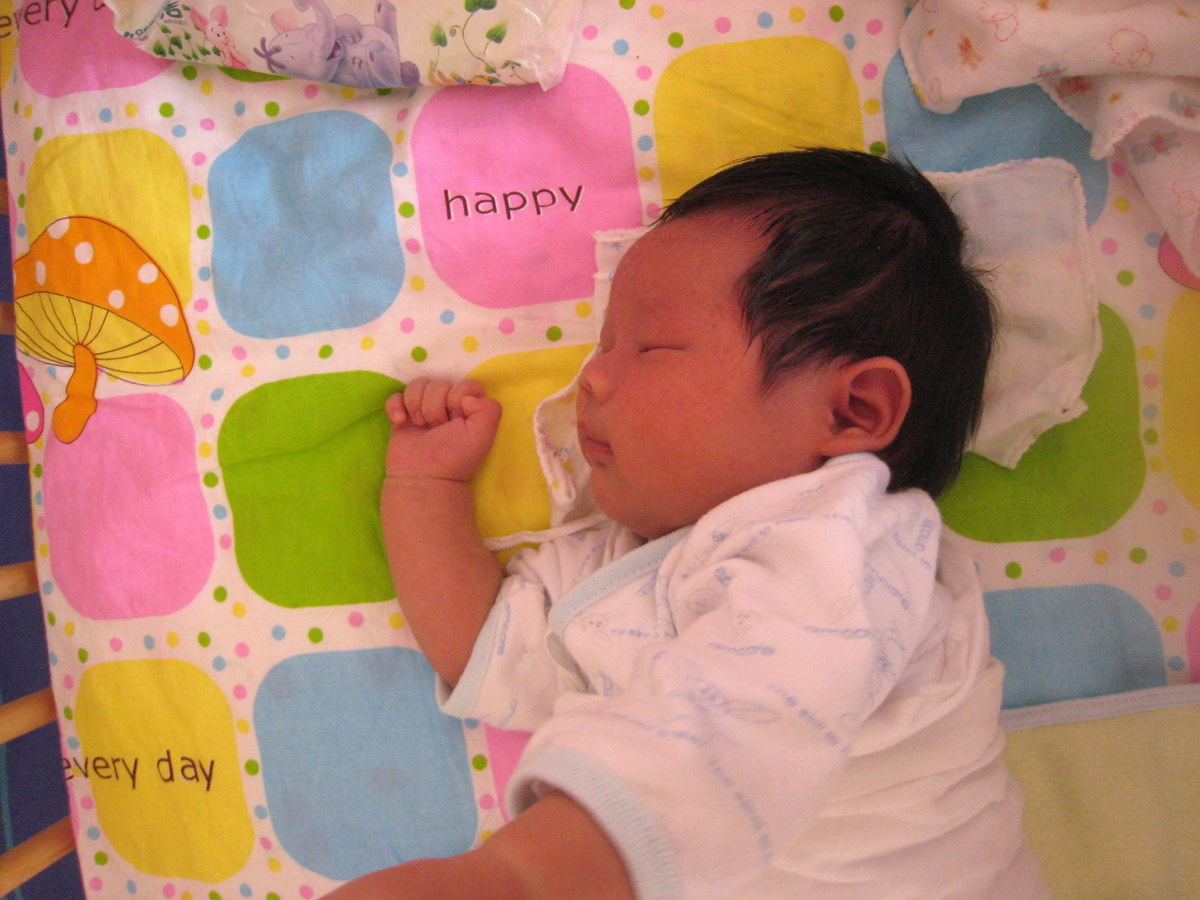This image showcases a serene baby with medium-length dark black hair, likely of Asian descent, peacefully resting on its side atop a vibrant, colorful blanket. The baby is dressed in a white onesie with baby blue trim along the neck and sleeves. The blanket beneath the baby features an array of soft, circular objects in yellow, blue, pink, and green, with some circles encapsulating the larger ones. One of the pink circles is inscribed with the word "happy." The blanket also includes illustrations of an orange mushroom and the inspiring phrase "every day" in the bottom left corner. The photo is taken from a top-down perspective, capturing the cozy ambiance of the indoor setting.